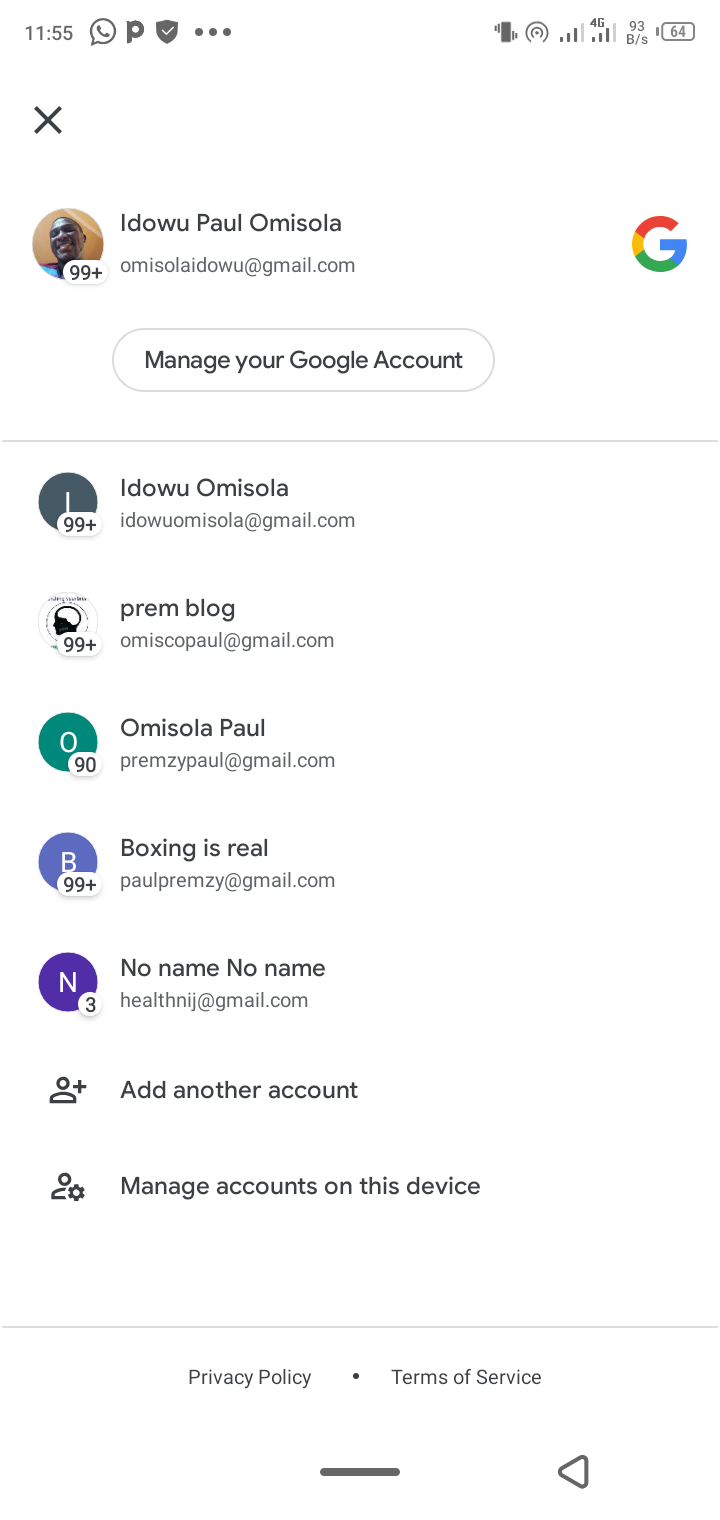This detailed description provides insight into an interaction with a Google account management interface on a mobile device. Here is a cleaner, more structured caption:

---

This vertical rectangular image, captured from a smartphone, showcases the Google account management screen. Across the top border, there is a status bar displaying the time as 11:55 in black text. Adjacent to the time are several icons including a phone, a "P" symbol, a shield, and three horizontal dots, indicating various service states and options. 

On the right side of the status bar, a vibrate mode icon appears next to a series of concentric circles with an opening at the bottom, indicating notifications. To the left of the circles are two signal strength bars and a battery icon showing a 64% charge. Below this interface, a small "X" appears.

The central portion of the screen features a prominent circular user profile image of a Black man with the name "Iduwo Paul Omisola" displayed next to it. His email address is listed below his name. To the right of the profile information is the Google "G" icon. Beneath this, an oblong box captioned "Manage your Google Account" dominates the scene, followed by a list of linked Gmail addresses.

Further down, options to "Add another account" and "Manage accounts on this device" are presented. These sections are separated by a thin gray line from the "Privacy and Terms of Service" section at the bottom. Each portion captures the detailed and organized structure of the Google account management interface on a smartphone.

---

This detailed caption should accurately convey the specifics of the image's content and layout in an organized and clear manner.